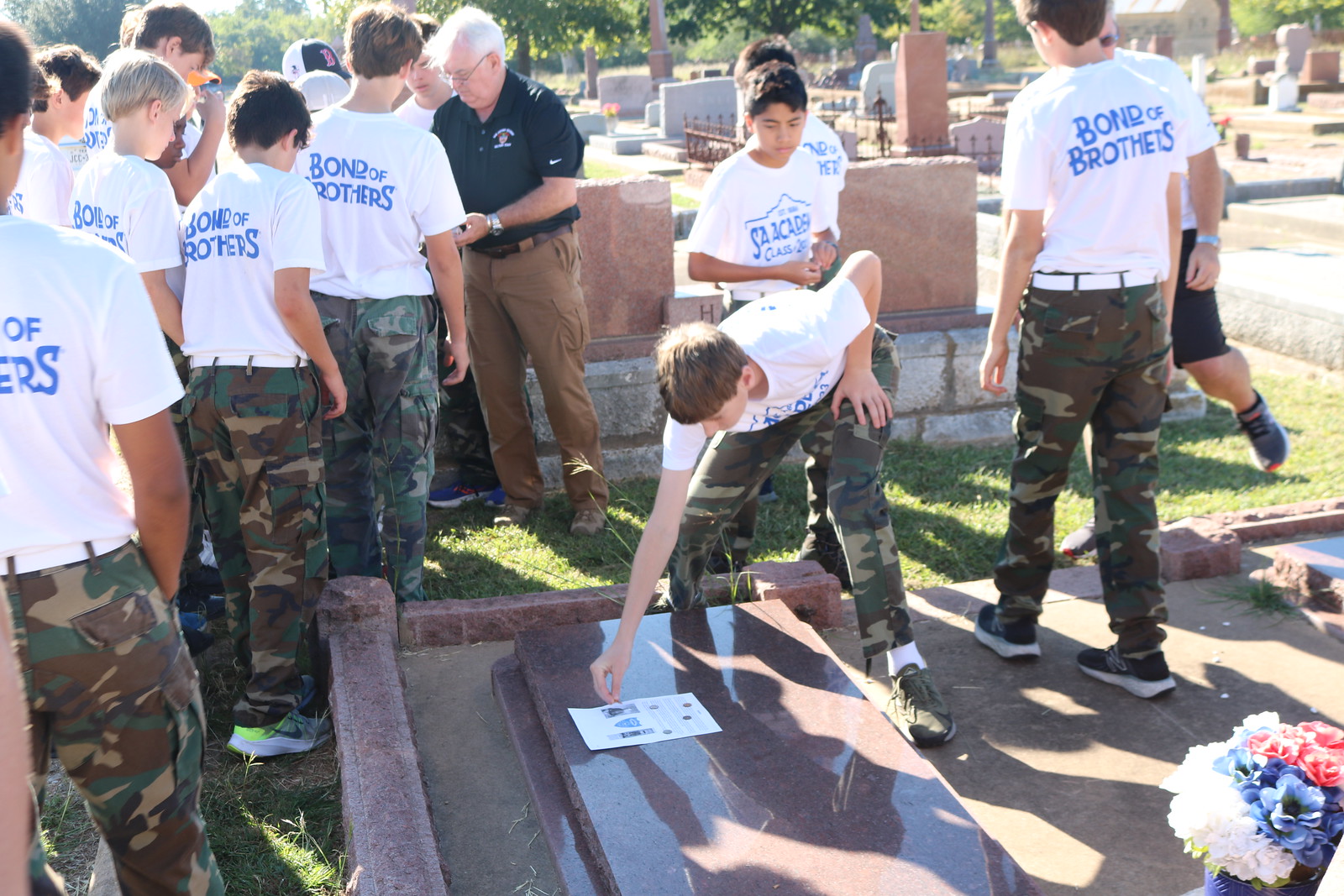This image depicts a group of young volunteers, likely Junior ROTC students based on their camouflage pants and white t-shirts emblazoned with "Bond of Brothers" in blue letters. They are gathered in a graveyard with numerous headstones, including a notably shiny red marble headstone lying flat at the bottom of the image. The students are lined up, seemingly engaged in an activity such as placing flowers—which are visible in blue, soft red, and white—on the graves as part of a charitable function. Among them, one boy in the center is bent over a flat headstone, possibly attaching a notice or tribute. Overseeing them is an adult with gray hair, dark-framed glasses, a black short-sleeved collared shirt, khaki pants, and brown shoes. The surrounding grass and late-day sunlight casting shadows on the ground create a serene yet purposeful atmosphere in the cemetery.